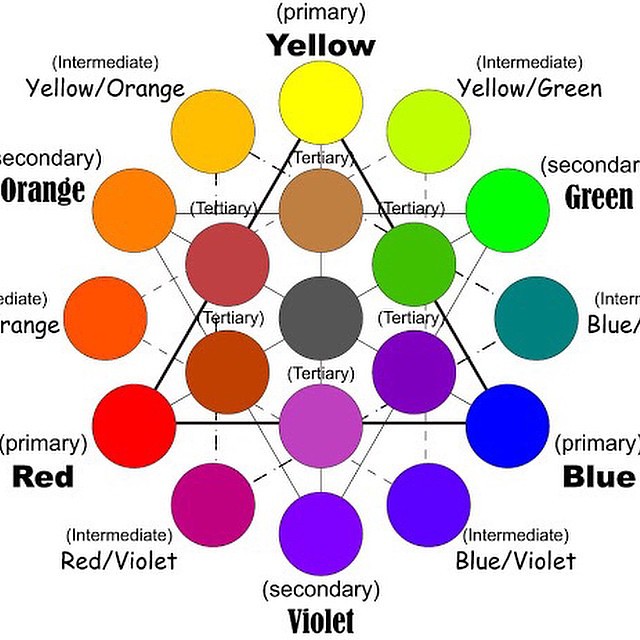The image is a detailed color wheel chart set against a white background. At the center is a black triangle from which black lines radiate outward, connecting to various colored circles. These circles represent primary, secondary, and intermediate colors, with black letters denoting each hue. Starting from the top and moving clockwise, the chart displays yellow (primary), yellow-green (intermediate), green (secondary), blue-green (intermediate), blue (primary), blue-violet (intermediate), violet (secondary), red-violet (intermediate), red (primary), red-orange (intermediate), orange (secondary), and yellow-orange (intermediate). Enclosed within these outer circles is another ring of colors labeled as tertiary, featuring shades such as brown, green, purple, light purple, reddish-brown, and purplish-brown. At the very center of the wheel, a gray circle is also marked as tertiary. This structured layout of primary, secondary, and tertiary colors mimics the kind found in school art classes or textbooks, providing a clear visual representation of color relationships.